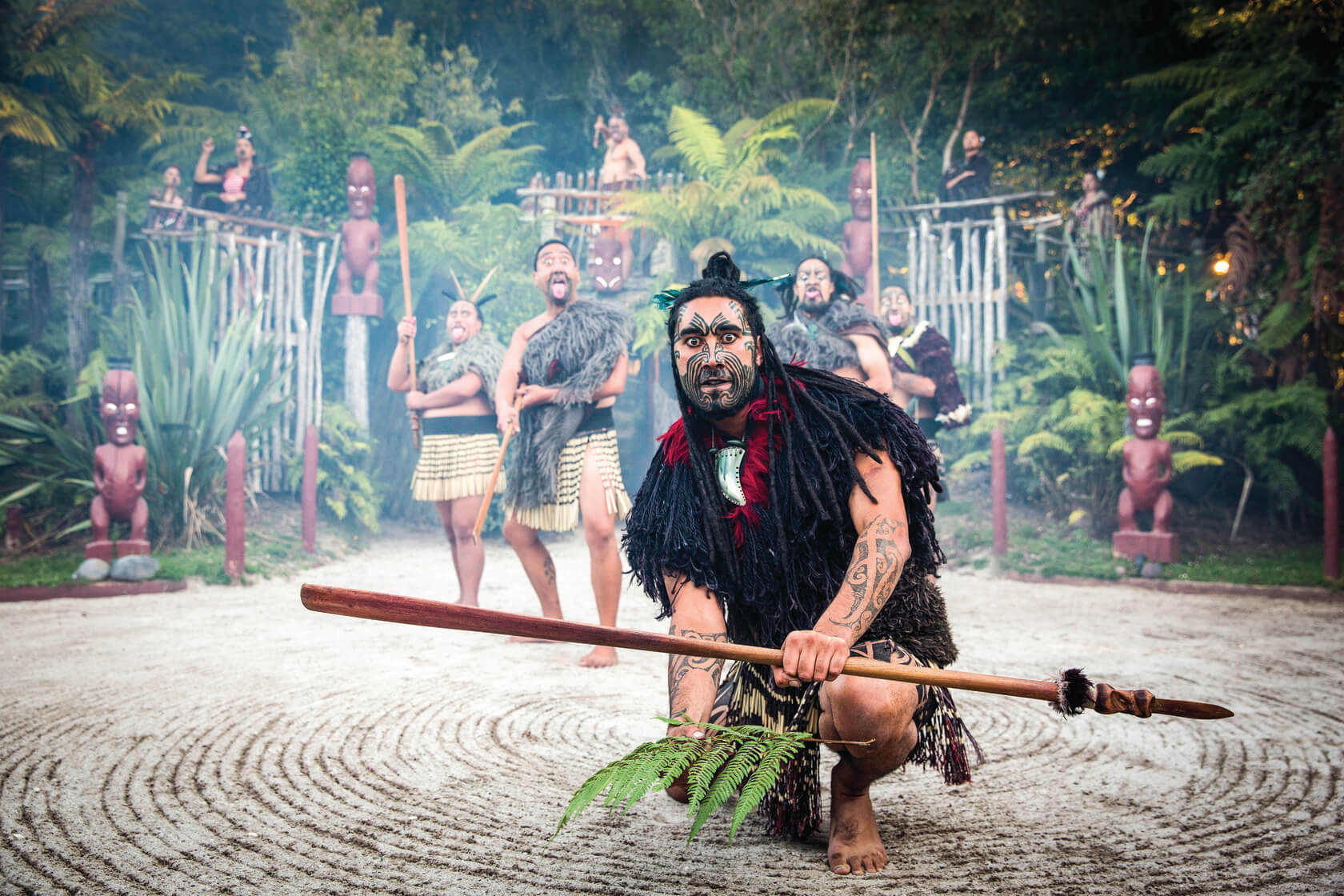In this vibrant outdoor setting, a man takes center stage, kneeling on one knee amidst a gathering of individuals dressed in indigenous, tribal costumes. His warrior makeup and intricate tattoos complement his dreadlocks, while he wields a large spear and a green palm or fern frond in his hands. Surrounding him, other men, possibly of African or Native American descent, are clad in grass skirts, shawls, and wield spears, with some exuding playful expressions. The backdrop is rich with tropical foliage, tiki statues, and wooden bamboo poles, suggesting a lively tribal performance. The scene is set on a distinctive circular, stone-like platform, evoking memories of cultural exhibitions, such as those at the Polynesian Cultural Center in Hawaii.